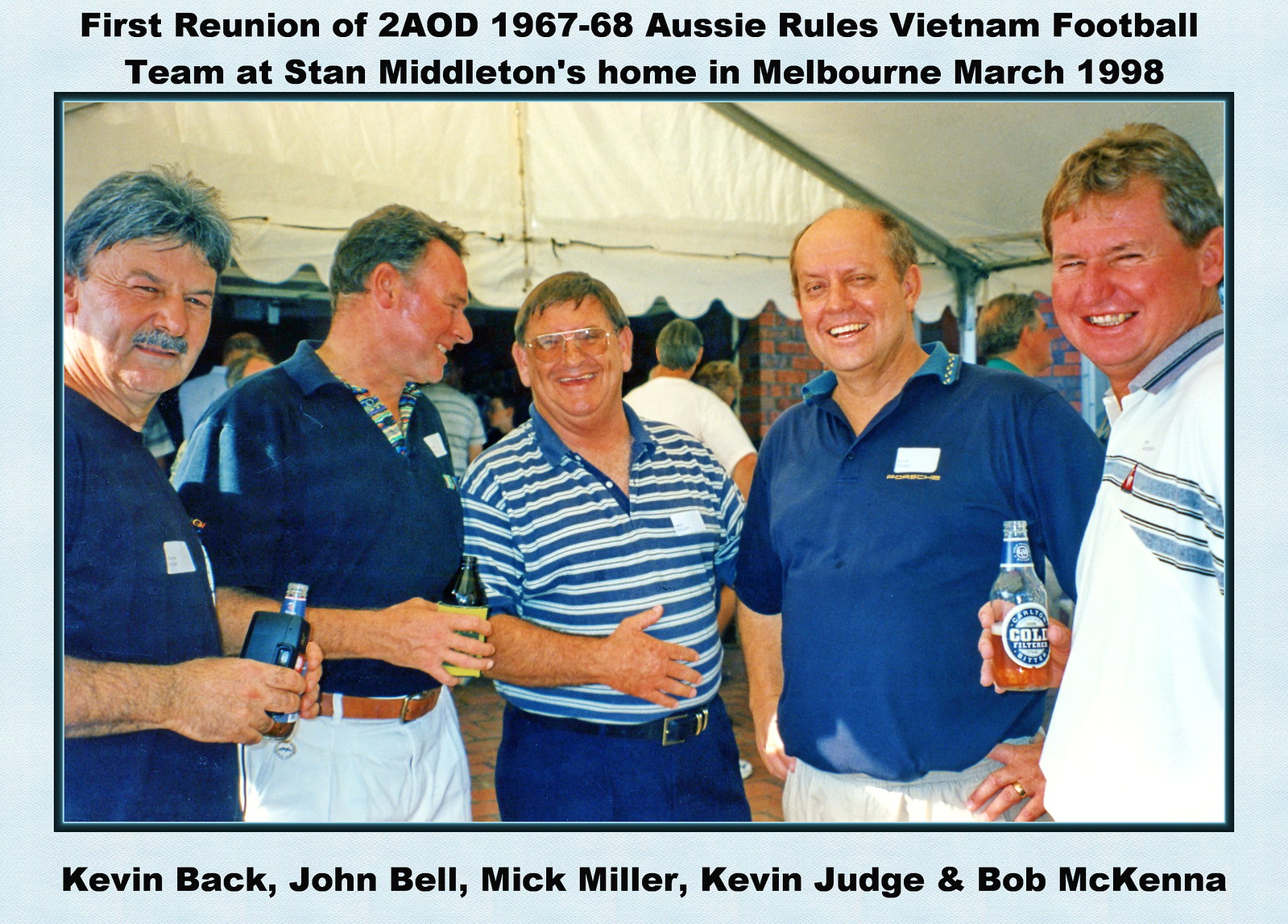The photograph captures a joyful reunion of five men, identified as Kevin Beck, John Bell, Mick Miller, Kevin Judge, and Bob McKenna, held at Stan Middleton's home in Melbourne in March 1998. The occasion marks the first reunion of the 1967-68 Aussie Rules Vietnam Football Team (Two AOD). The image is enclosed within a decorative frame featuring a light blue border with a darker blue inner trim. The border at the top displays the event details and the participants' names are listed at the bottom in black font. 

Set under a white canopy tent, the five men stand out despite the bustling background. They are all dressed in variations of blue and white attire. The man on the far left, with a gray mustache, holds an old-style box vape machine and a green beer bottle. The man next to him wears a solid blue polo shirt and white pants, clutching a similar green beer bottle with a yellow label identified as Carlton Bitter. The central figure dons a blue and white striped shirt. The man to his left, slightly balding, is also in blue. The far-right individual sports a white shirt with blue stripes and glasses, holding the same kind of beer bottle as the man on the far left. The group all smiles at the camera, clearly enjoying their time together at this nostalgic event.